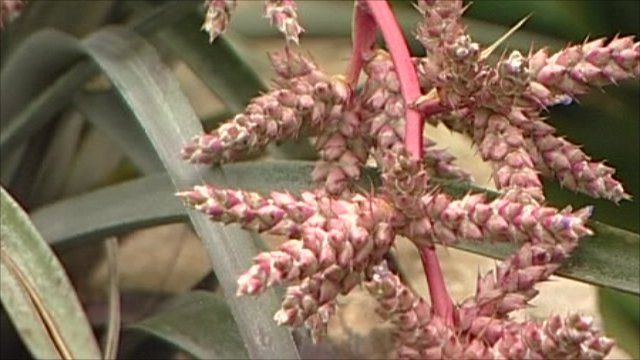This image features a close-up of a distinctive plant that appears to have both cactus and thistle-like characteristics. Dominating the center is a long, drooping stem in a darker pinkish-red hue, which thickly sprouts dense clusters of rounded pink and white buds, resembling acorns or cola buds. These buds are bound together and connected by a central pink rod or handle. Surrounding the primary plant are tall, narrow, olive-green leaves that extend vertically and diagonally, some even cutting through the main pink structure. This lush backdrop of green foliage, with leaves resembling those of succulent plants, adds to the jungle-like ambiance. The overall visual is somewhat digitally zoomed, with noticeable compression affecting image clarity.